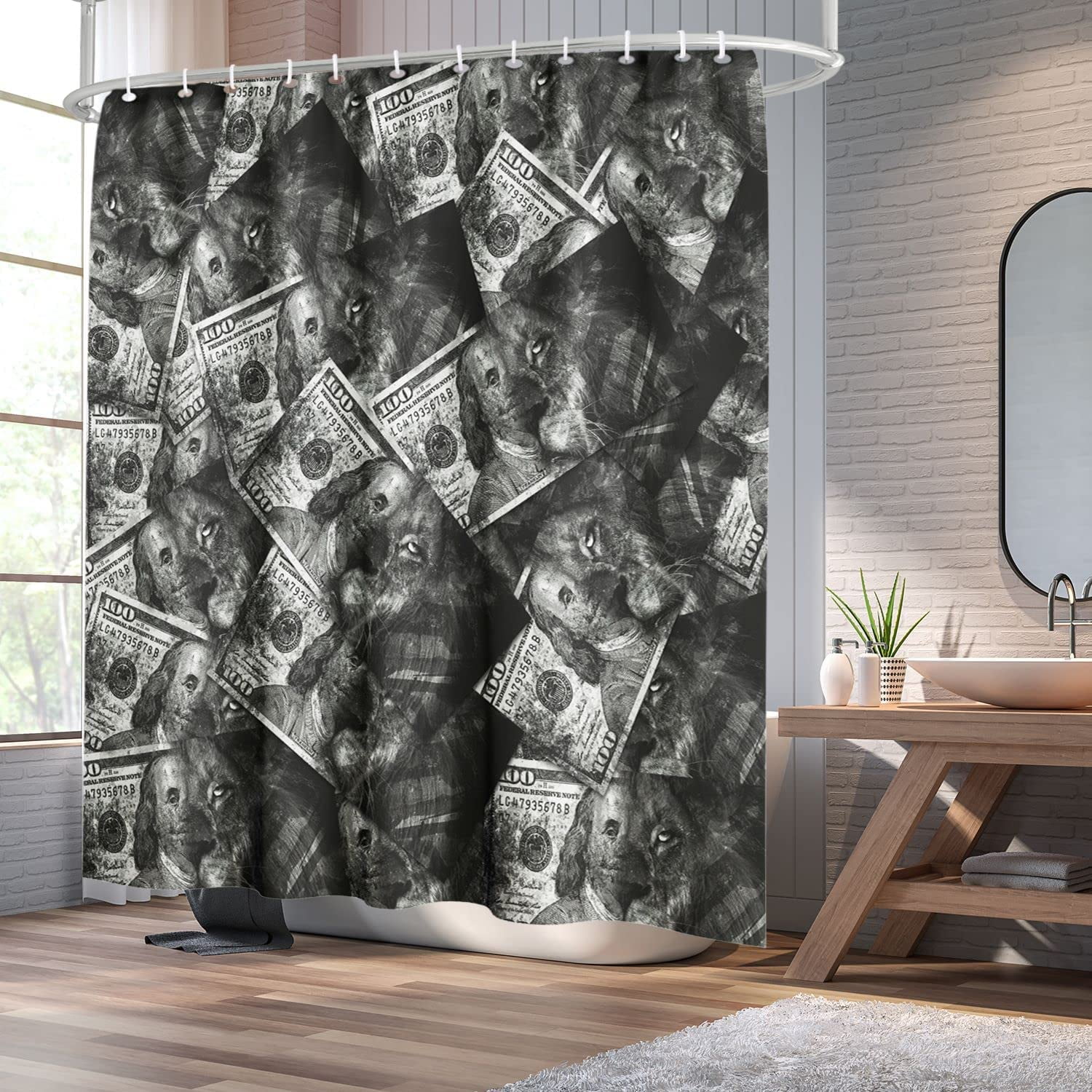This photograph captures a stylish and unique bathroom setting. The focal point is a striking grayscale shower curtain adorned with an intriguing print of $100 bills interwoven with the face of a lion. The bathroom features light hardwood floors and a fluffy gray carpet mat. On the right-hand side, there's a long oblong mirror mounted on a beige brick wall. The sink is a white ceramic bowl set on a light brown wooden stand with a single shelf underneath holding gray towels. Atop the stand are pumps likely for soap or shampoo. Additionally, a desert aloe vera plant in a white pottery planter adds a touch of greenery. On the left, there is a large window allowing natural light to flood in, enhancing the overall aesthetic of this meticulously decorated space.